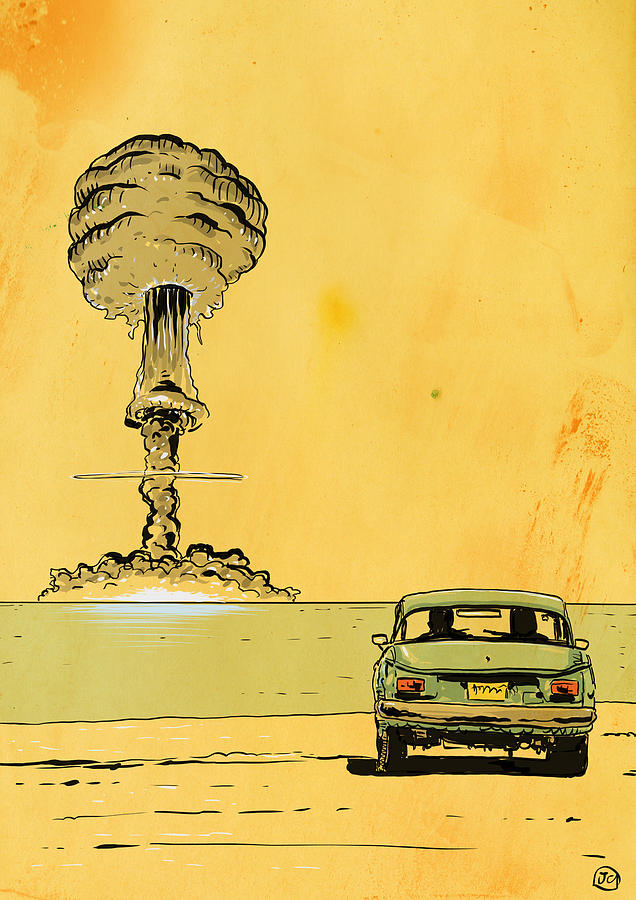This colored illustration, predominantly in shades of yellow, depicts a vivid post-apocalyptic scene. In the foreground, a light green, 1950s steel-body car with red taillights is parked, its back facing the viewer. Two figures are visible inside the car, gazing forward at the dramatic sight before them. The setting appears to be a flat, possibly beach-like, area with slight reflections of light on an adjacent body of water. Dominating the background is an immense mushroom cloud, the result of a nuclear explosion, rising tall on the horizon. The cloud is an olive-green hue, contrasting with the bright yellow and peach-colored background. Above the car, a streak of red extends upward and to the right, adding to the intense atmosphere. At the very bottom of the image sits the artist's signature — a drawn circle with the letters "J O" inside.